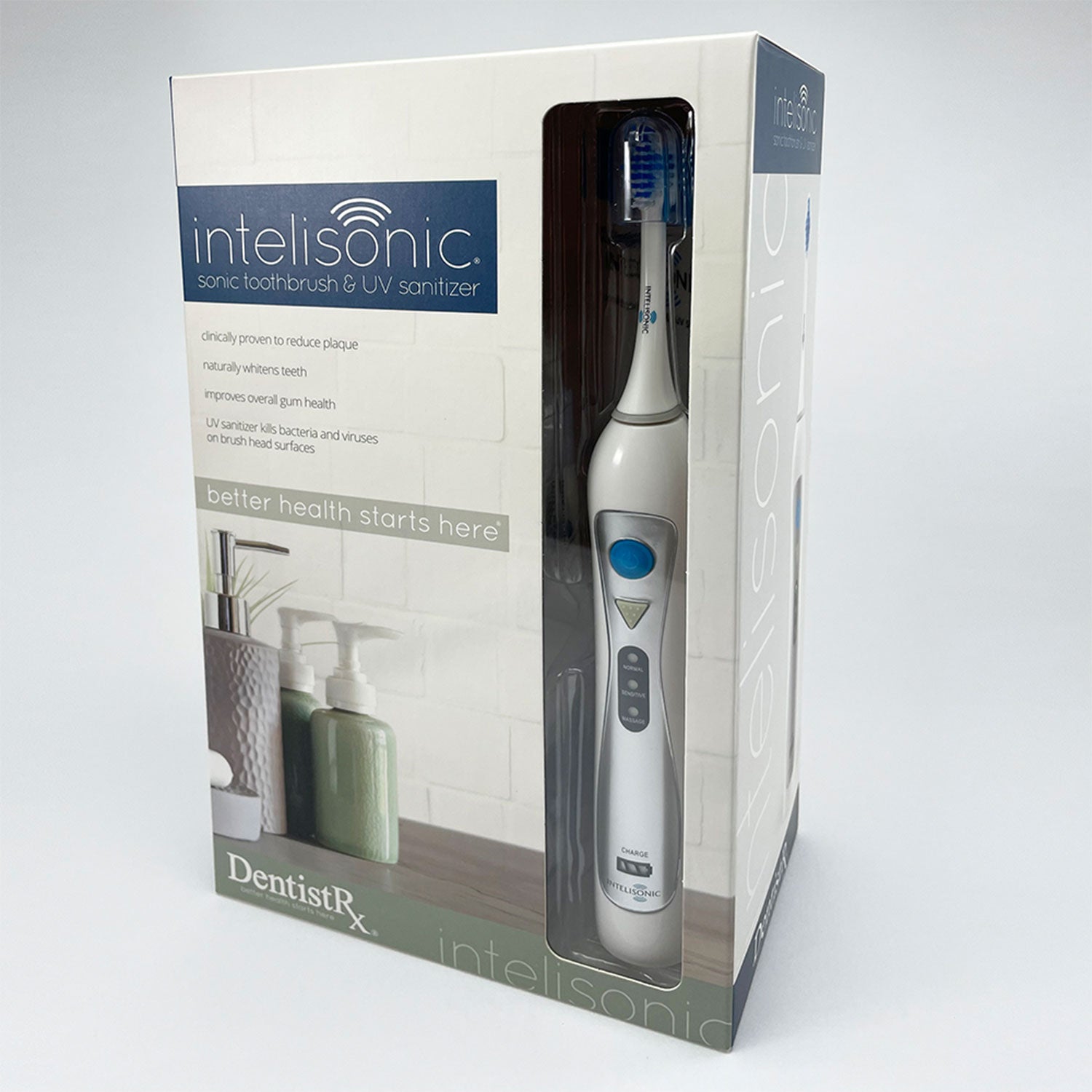This is a detailed, professional photograph of an Intellisonic Sonic Toothbrush and UV Sanitizer, displayed against a clean, white-beige background. The toothbrush is still inside its unopened beige and white box, which features a transparent plastic window allowing visibility of the toothbrush. The toothbrush itself is approximately 8 inches tall, predominantly white with blue buttons and a blue head. Prominently displayed on the box is a blue text bar with white writing that reads, "Intellisonic Sonic Toothbrush and UV Sanitizer." Just below this, in bold, it states the tagline, "Better Health Starts Here." The box also contains a small image depicting a bathroom scene with hand soaps, emphasizing its appropriate placement in a home setting. Additional small print on the box highlights the toothbrush's benefits, including plaque reduction, teeth whitening, and improved gum health.